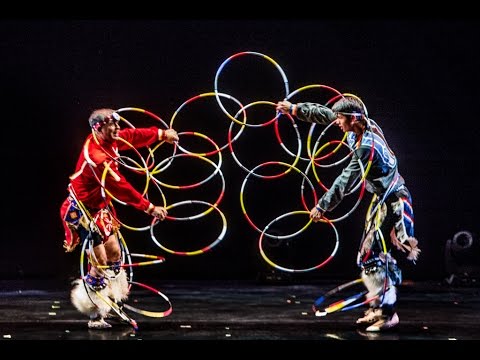This image captures two performers in vibrant attire on a dark stage, suggesting they are engaged in a carefully coordinated act. The older man on the left wears a red sports jacket adorned with intricate beading and fur-trimmed boots, complemented by what appears to be a headlight on his head. Opposite him stands a younger man in his late teens to mid-20s, donning a blue jacket with similar beading and fur boots. Both performers, who exude an aboriginal-inspired aura despite the modern elements of their costumes, hold an array of about twenty intertwined, multi-colored hula hoops. The hoops, encompassing hues of blue, red, yellow, white, and purple, loop and arch around their bodies, connecting them in a mesmerizing display that stands out starkly against the all-black background and stage floor.